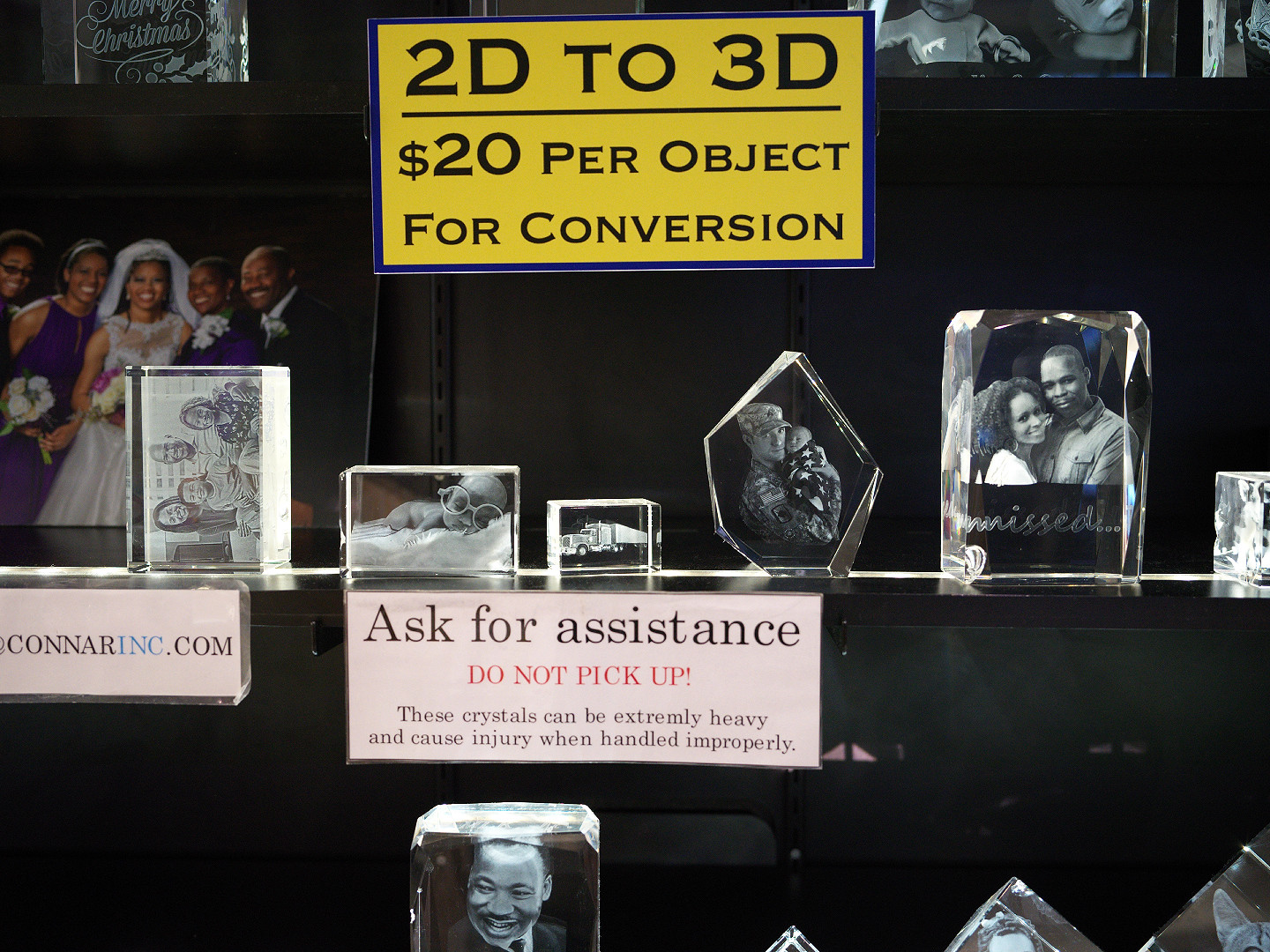The image depicts a store display featuring a selection of clear crystal ornaments etched with various images, arranged on black shelving against black walls. At the top center, a bright yellow sign with a blue border and black text reads: "2D to 3D. $20 per object for conversion." This indicates that you can convert a photograph into a three-dimensional etching within the crystals, which come in various shapes. The crystals display diverse scenes, including smiling families, babies, trucks, soldiers holding babies, couples, and a depiction of Martin Luther King Jr. A smaller pinkish-white sign below advises: "Ask for assistance. Do not pick up." The text warns that the crystals can be extremely heavy and might cause injury if handled improperly, with "Do not pick up" emphasized in red. Additionally, a partially visible website, "ConRInc.com," is noted on a sign to the side.